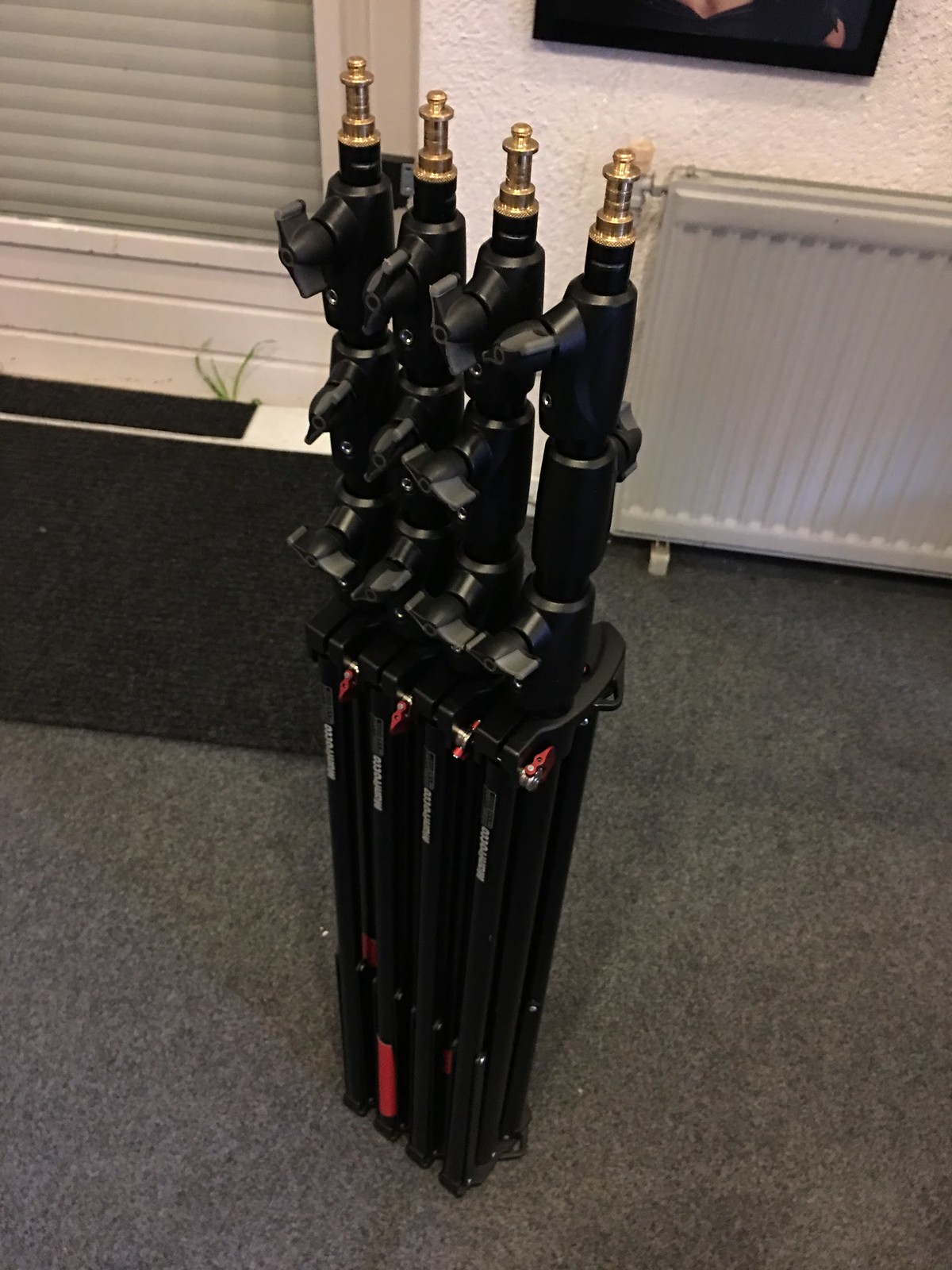The photograph captures a room with four vertically aligned folded tripods standing side by side on a dark grey, shaggy carpet. Each tripod features a gold metal tip at the top, a black plastic body, and various knobs and connectors for adjustments. The room's backdrop includes a white-paneled door with horizontal white blinds covering its window, nearly obscuring the view behind it. To the right, a white wall showcases a black-framed picture and a wall heater. Scattered red elements are visible among the tripods' connections, and a fabric floor mat lies in front of the door, adding to the detailed interior setting.